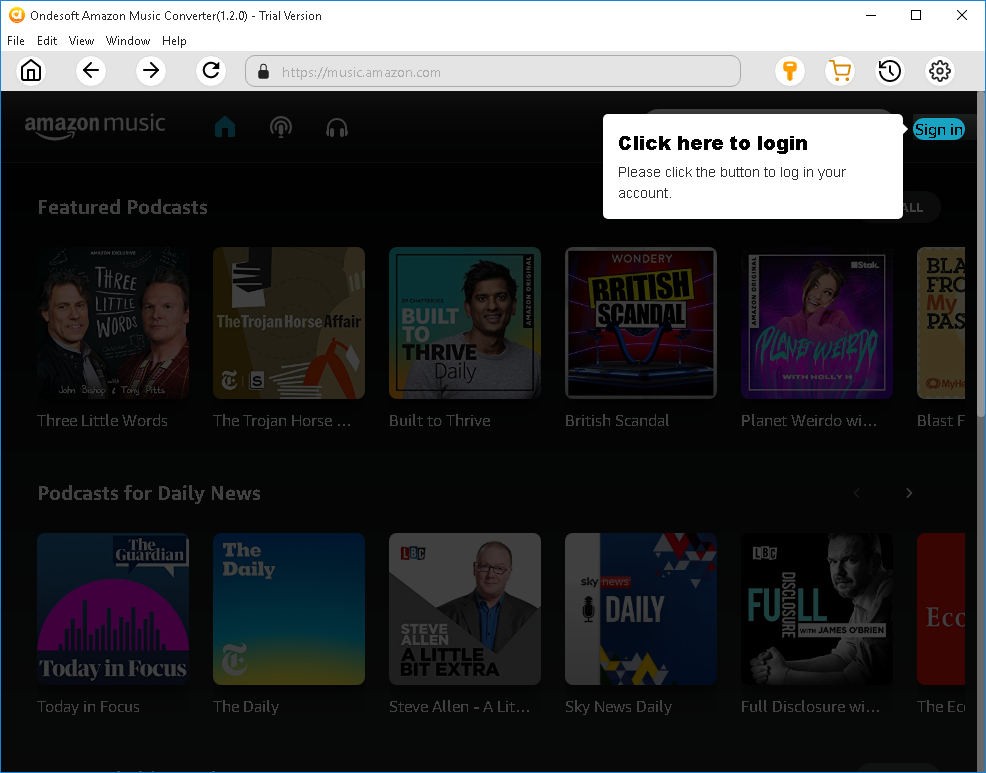In this image, we see a screenshot taken from an application or website. At the top in the title bar, there is an orange icon with a white "A" on it, indicating the software "OndaSoft Amazon Music Converter 1.2.0 Trial Version." To the right of this, we see the minimize, window, and close buttons. Just underneath, we find the typical menu options: "File," "Edit," "View," "Window," and "Help."

Below these menu options, there is a toolbar featuring several buttons: "Home," "Back," "Forward," and "Refresh." Next to these, there is a web address bar presently set to "https://music.amazon.com." Alongside the address bar, we see icons for a key, a cart, a clock with an arrow circling around it, and a settings gear.

The main content of the app displays the Amazon Music page, although it appears to be grayed out somewhat. Overlaid on the top right corner of this page, there is a pop-up message that reads, "Click here to log in. Please click the button to log in to your account," with an arrow pointing to a "Sign In" button.

Within the Amazon Music interface, we can spot the Amazon Music logo, icons for "Home," "Headphones," and "Broadcast." Below these, there's a section titled "Featured Podcasts," with a horizontal scroll of various podcast options. Further down, there is another section for "Podcasts for Daily News."